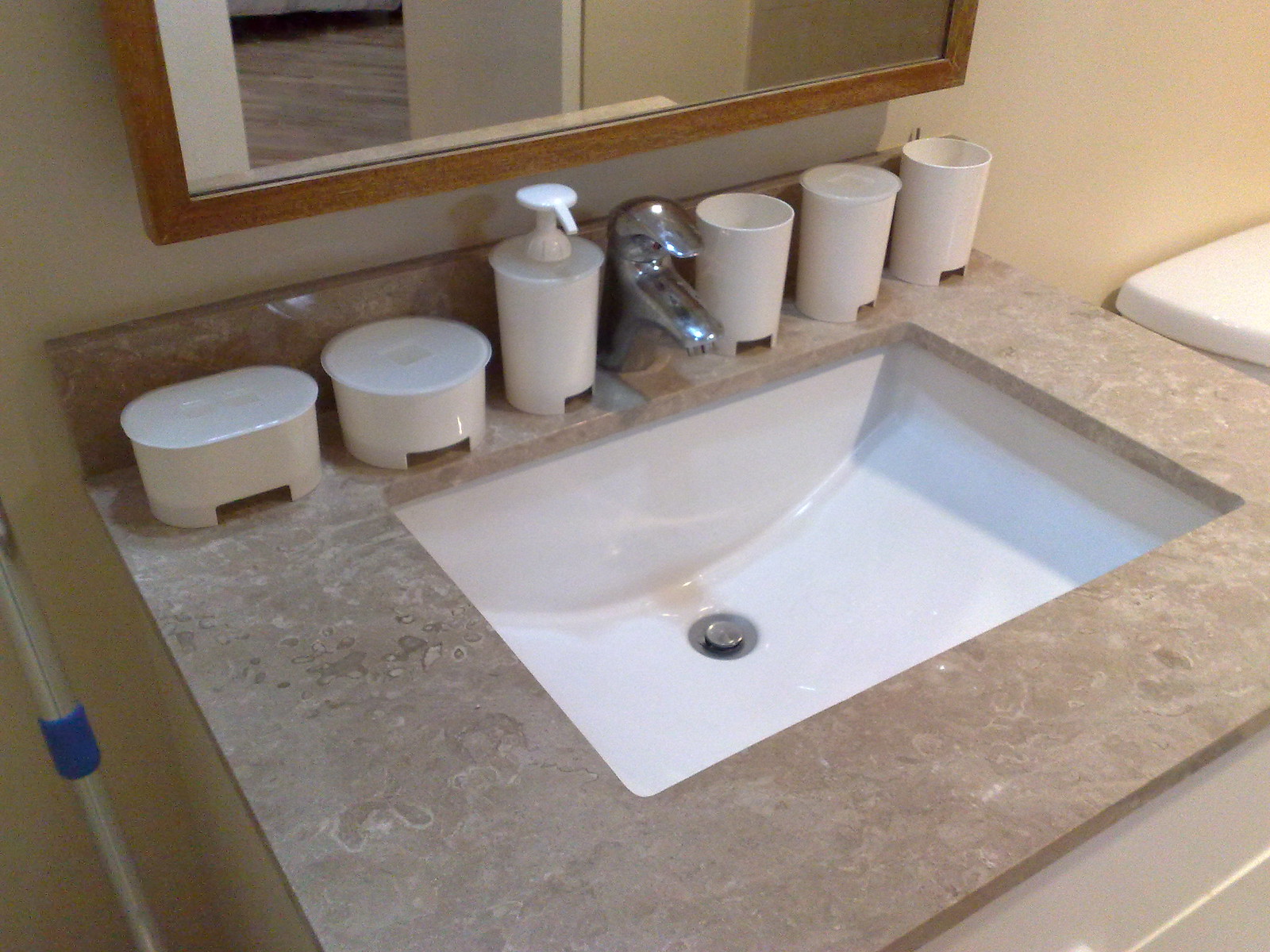This photograph captures a well-organized and clean bathroom. In the bottom right-hand corner, partially cut off, is a white cabinet situated beneath the countertop, matching the pristine white ceramic basin with a silver stopper. The countertop is a light brown marble with subtle swirls and gradients of gray and white. 

A stainless steel faucet complements the basin, with three white containers neatly arranged in a plastic holder immediately to the right. The second container from the left within this holder has a plastic lid. To the left of the faucet, another white plastic container stands upright, featuring a pump lid for dispensing soap. Adjacent to it are two more plastic containers, one circular and one oval, likely serving as soap dishes.

A silver handle with a blue plastic piece, possibly belonging to a mop or broom, is visible beside the sink. Above the countertop, a wooden frame with a light brown border houses a mirror, adding a touch of elegance to the bathroom's organized and clean aesthetic.